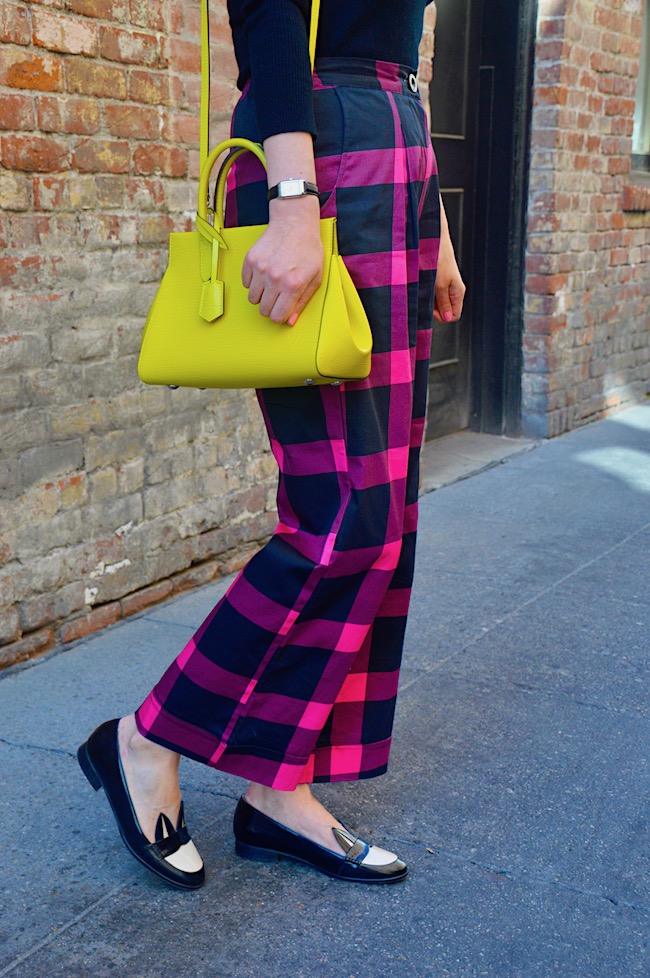The image captures a woman's lower half, showcasing her distinctive fashion. She wears vibrant, striped bell-bottom pants with hues alternating between pink, purple, and dark blue. The pants feature a brass button and are paired with black, slip-on shoes adorned with cat ear designs, revealing her feet slightly. She sports a bright yellow handbag slung over her right shoulder and a rectangular wristwatch on her left wrist. Her top is a long-sleeved, black shirt. The background displays a textured stone wall in orangish-brown shades with a black door, and she stands on a stone-tiled sidewalk that is blue-gray in color.